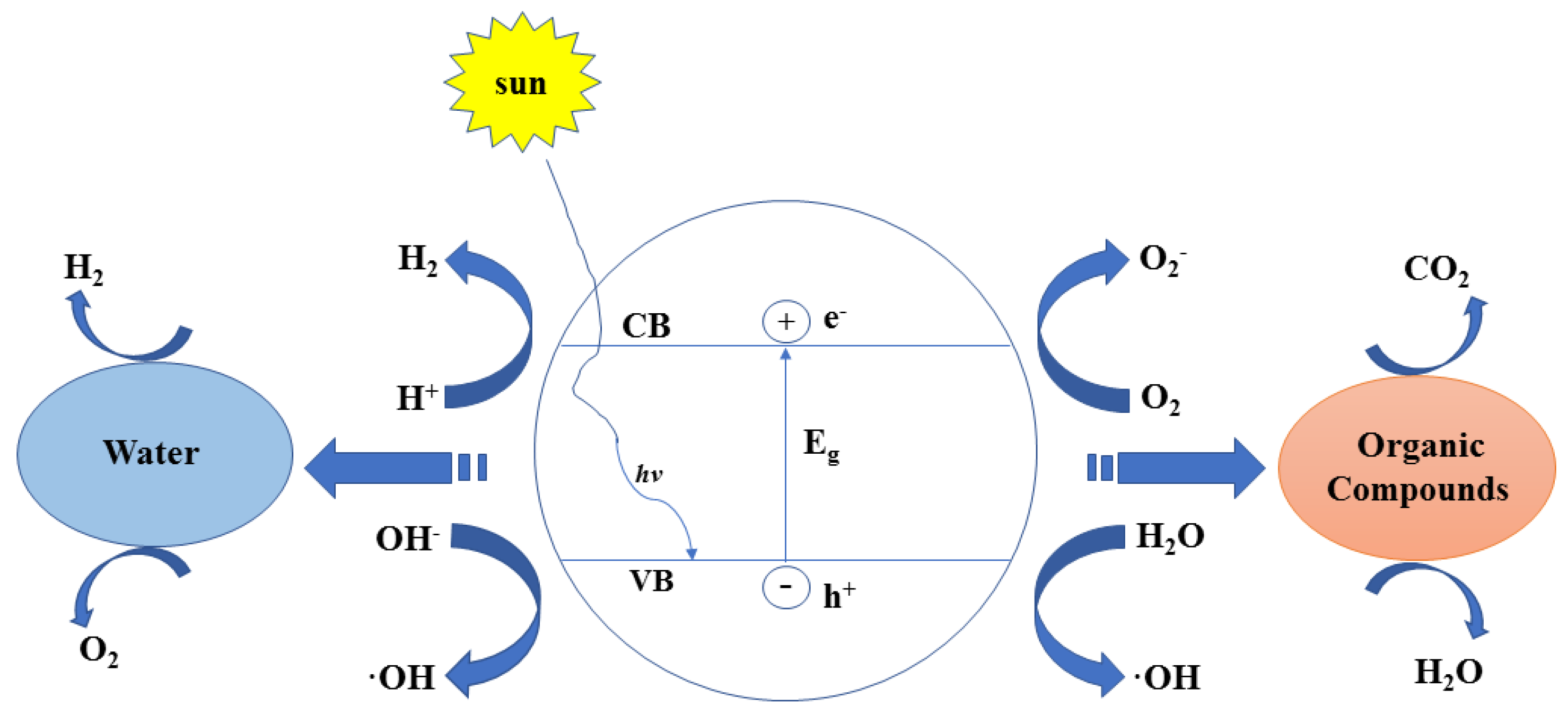Set against a white background, this detailed scientific diagram illustrates a complex chemical process. At the center is a large circle with a thin blue outline, within which various chemical symbols such as CB, VB, E, EG, H+, O, and O2 are displayed. Above and slightly to the left of this central circle is a yellow sun with the word "sun" inside it, from which a squiggly blue line descends into the large circle, indicating the entry point of sunlight into the process. On either side of the central circle are multiple arrows. To the left, blue arrows point from the central circle to a horizontal blue oval labeled "water," featuring chemical notations H2, H+, O2, and OH-. To the right, blue arrows extend from the central circle to a peach-colored oval labeled "organic compounds," containing notations like CO2 and H2O. The diagram collectively depicts the movement and transformation of elements and compounds, possibly illustrating a photosynthetic or chemical reaction process involving the conversion of carbon dioxide and water into organic compounds under the influence of sunlight.